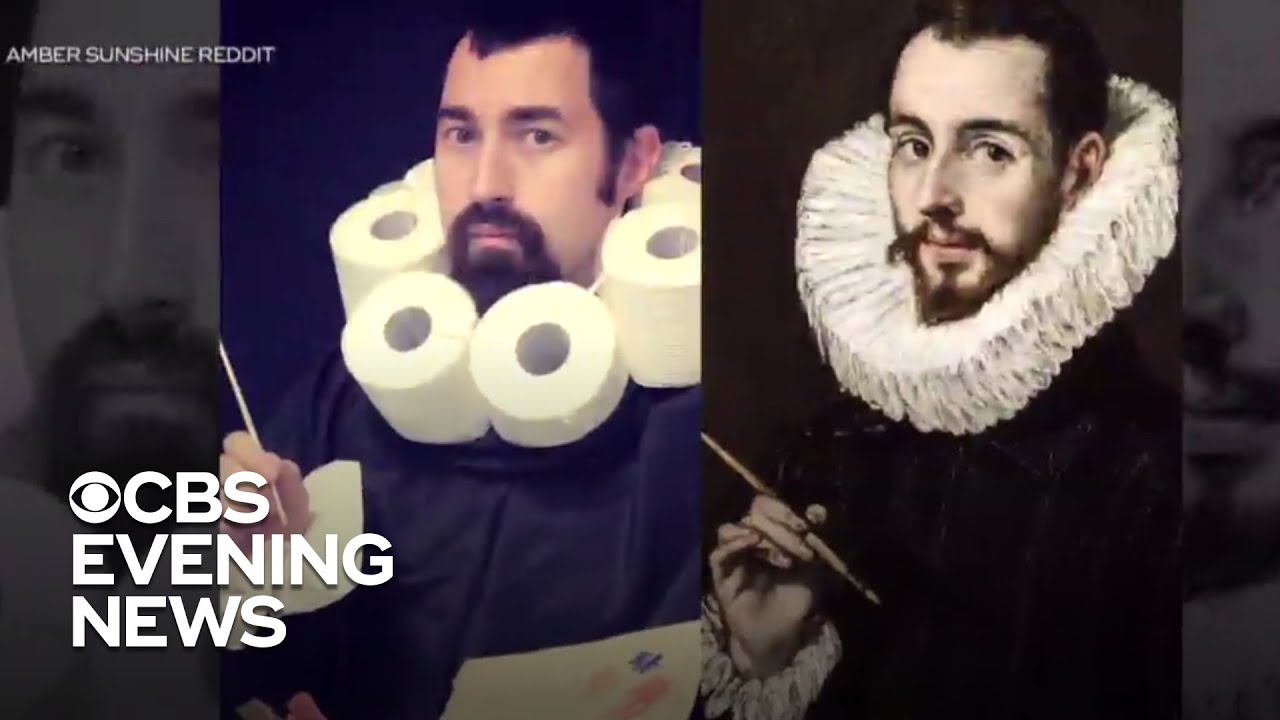This is a detailed visual description of a composite image comparing a modern-day gentleman with a classic portrait of William Shakespeare, framed as part of a screenshot from a news article. The upper left corner of the graphic displays "Amber Sunshine Reddit" in white text, while the lower left corner features the CBS Evening News logo and the words "CBS Evening News."

At the center of the photograph, a Caucasian man with dark hair, a goatee, and sideburns mimics the attire and pose of Shakespeare. He sports toilet paper rolls around his neck resembling a makeshift frilly collar, and wears a black jacket. In his right hand, he holds a paintbrush, and in his left hand, he appears to be holding a piece of toilet paper used as an artist's palette with paint blots visible on it.

Next to this modern man’s image is a classic black-and-white portrait of William Shakespeare, featuring similar dark hair, a white face, and a black goatee. Shakespeare is depicted wearing a traditional fluted collar and a black jacket, holding an artist's brush, mirroring the pose and elements of the modern photograph. The comparison highlights the parody and visual similarities between the two subjects.